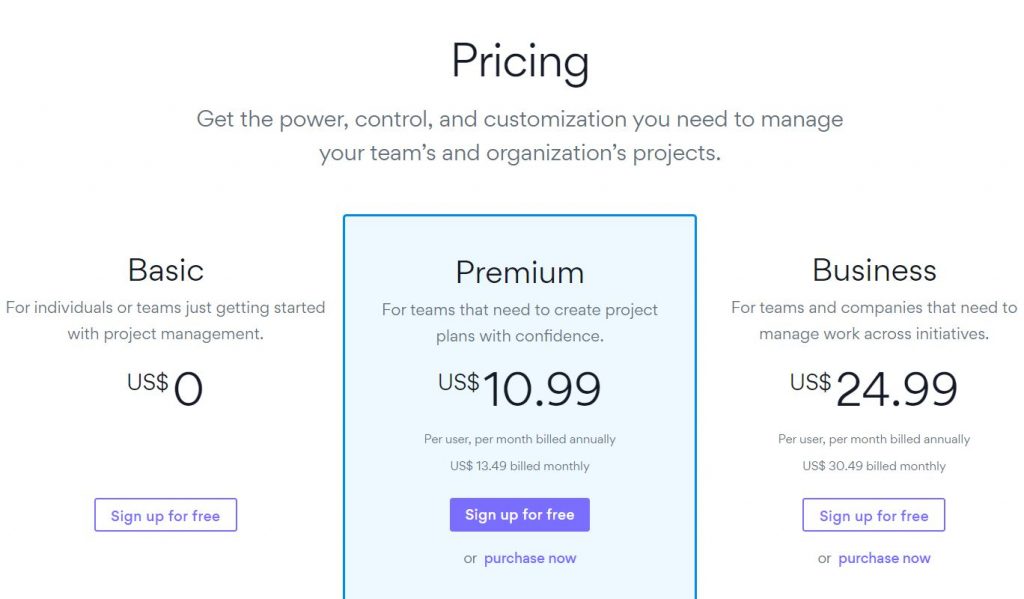A person is examining the pricing options for a subscription-based service. At the top of the display, the word "Pricing" is prominently featured. Beneath it, a caption reads, "Get the power, control, and customization you need to manage your team's and organization's projects." Below this, three subscription options are presented in a row. 

On the left, the "Basic" plan is designed for individuals or teams beginning with project management. This plan is free of charge, with an option to "Sign Up for Free" in a straightforward black font.

In the center, the "Premium" plan caters to teams that require confident project planning. It is priced at $10.99 per user per month when billed annually, or $13.49 per user per month when billed monthly. The "Premium" option is highlighted in blue, indicating it is selected. A prominent purple button allows users to "Sign Up for Free or Purchase Now."

On the right, the "Business" plan targets teams and companies needing to manage work across multiple initiatives. It costs $24.99 per user per month when billed annually, or $30.49 per user per month when billed monthly. This plan also features a purple button offering the choice to "Sign Up for Free or Purchase Now."

The entire interface sports a clean design with a white background, simple black text, and purple accents for hyperlinks and buttons. The font used is uncomplicated and easy to read, ensuring clarity throughout.